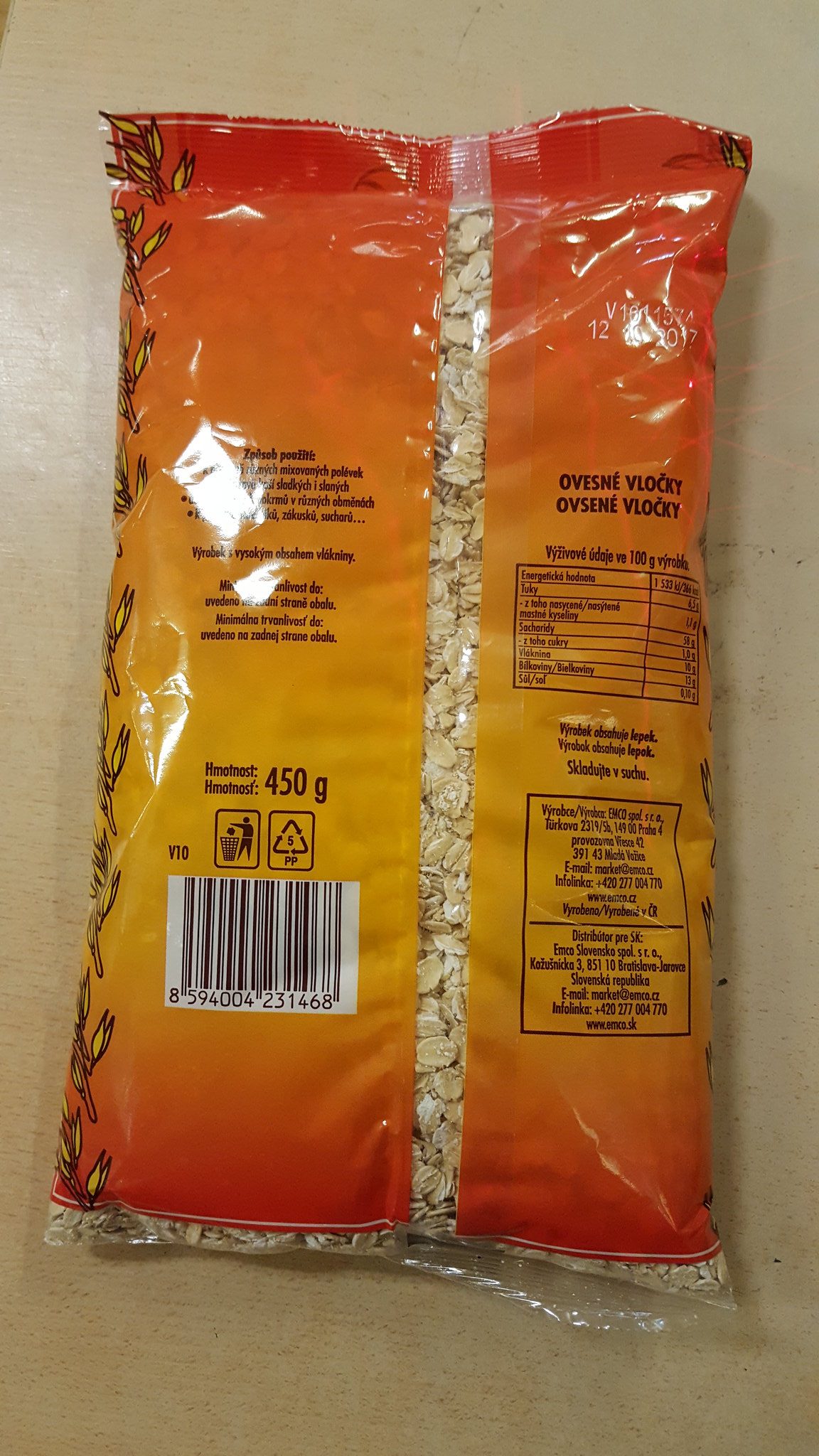This is a photograph of the back of a processed food package, likely containing rolled oats or similar grains. The package features a vibrant ombre effect transitioning from yellow in the middle to darker orange and red at the edges. A clear strip runs vertically down the center, allowing the contents to be visible. The packaging includes numerous labels and text in a foreign, likely European, language. The left side shows yellow leaves on an orange stalk, with black text that might be in Polish and mentions "HMOT NOST 450 grams". The bottom left corner features a barcode with the number 8594004231468. The recyclable plastic icon and a '5' recycling code are also present. The nutritional label is situated on the right side, mentioning the Republic of Slovenska. The entire package rests on a very light, brownish wooden or possibly linoleum surface.